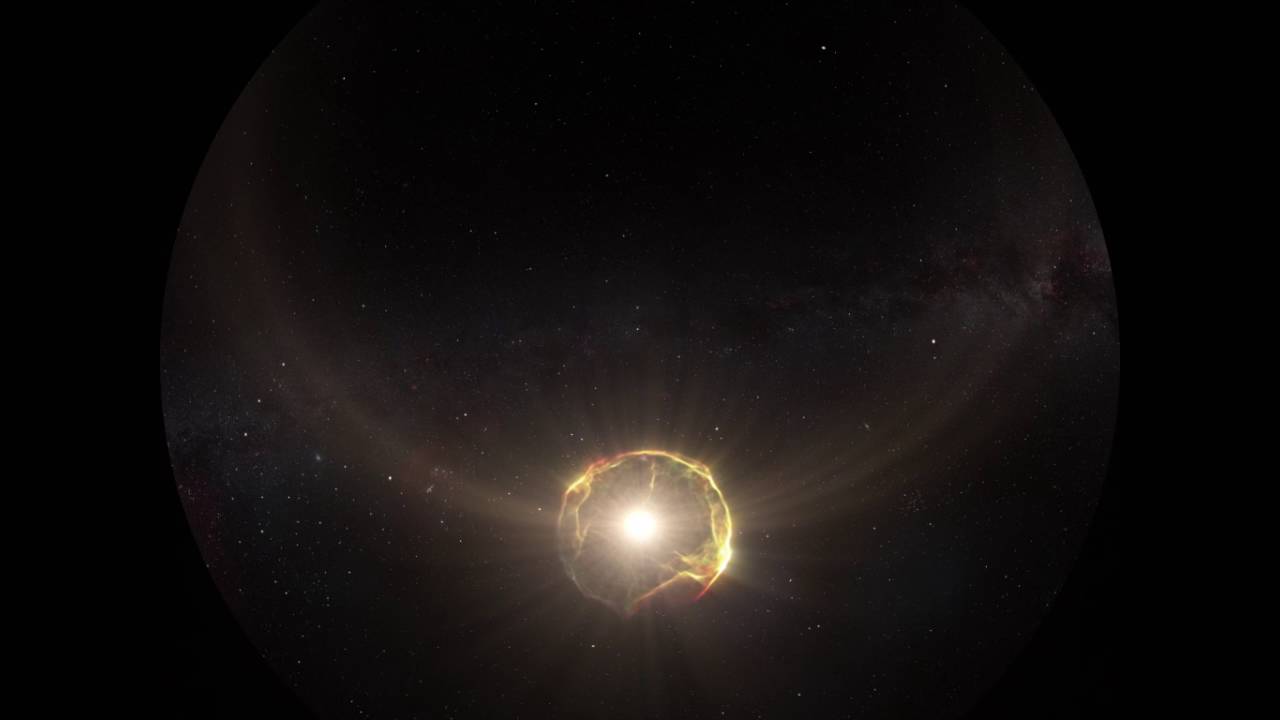The image captures a dark, almost black night sky filled with an array of stars, some bright and others dim. Dominating the bottom center of the image is a brilliant and radiant moon, which exudes a bright, whitish light with a halo-like glow that imparts an almost angelic appearance. This luminous sphere is surrounded by colors that range from bright white to golden yellow, creating an ethereal, reflective globe effect. The surrounding sky is a mix of deep black with streaks and hints of gray. There are also streaks of orange, red, and gold scattered across, giving the impression of a hyper-realistic portrayal, possibly taken with a telescope. The vivid, glowing lines curving upward and outwards from the moon enhance the celestial beauty of the scene, making it appear as a captivating blend of reality and artistic interpretation.